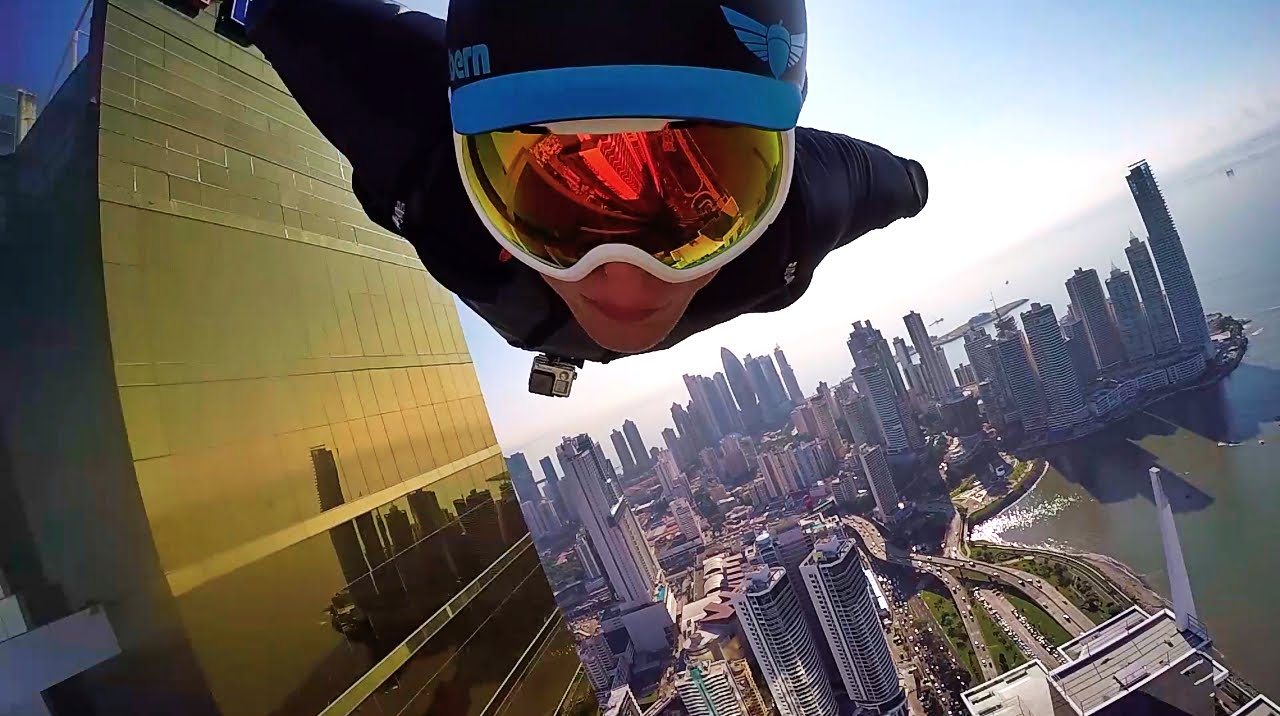This photograph captures a thrilling selfie taken by a parachuter or hang glider during their descent from a skyscraper, likely in a city such as Chicago or New York. The individual, who appears to be female based on facial features, is wearing distinctive blue and black gear, including a helmet, blue goggles tinged with yellow and shades of red, and a black jacket with a prominent metal fixture on the front. Although the helmet bears letters that spell out "E R N A" with the remainder obscured, there are no other identifiable markings. The image's composition is striking, with the horizon tilted at a 45-degree angle, giving a dynamic sense of movement. Below, the aerial view reveals a bustling cityscape filled with towering buildings. Skyscrapers, including a twin-tower structure, dot the background on the right, while a large brown building from which the person likely jumped is prominently featured on the left. The lower part of the frame offers a glimpse of what might be an ocean, enhancing the dramatic context of the shot. The photograph's overall perspective is slightly warped, possibly due to the motion and the high altitude at which it was taken.